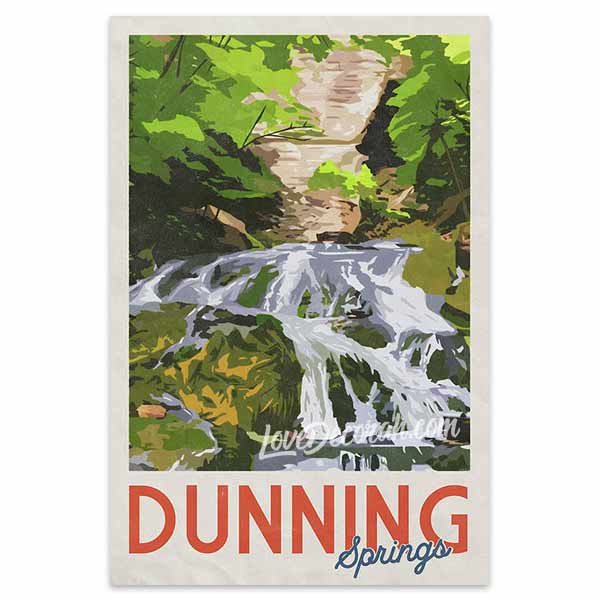The image is a poster featuring an acrylic-style illustration of a natural landscape. It displays a rocky waterfall, flowing into a larger pool of water, surrounded by green leafy trees. The sky at the top has subtle pink hues, giving a hint of early morning or late evening. The title "Dunning Springs" is prominently written across the bottom, with "Dunning" in bold red uppercase letters and "Springs" in blue with a white border. On the lower right corner, there is a watermark that reads "Lovedecorah.com," likely indicating a location or promotional website. The overall effect is a harmonious blend of natural elements and marketing, capturing the serene beauty of Dunning Springs in a detailed and vibrant manner.